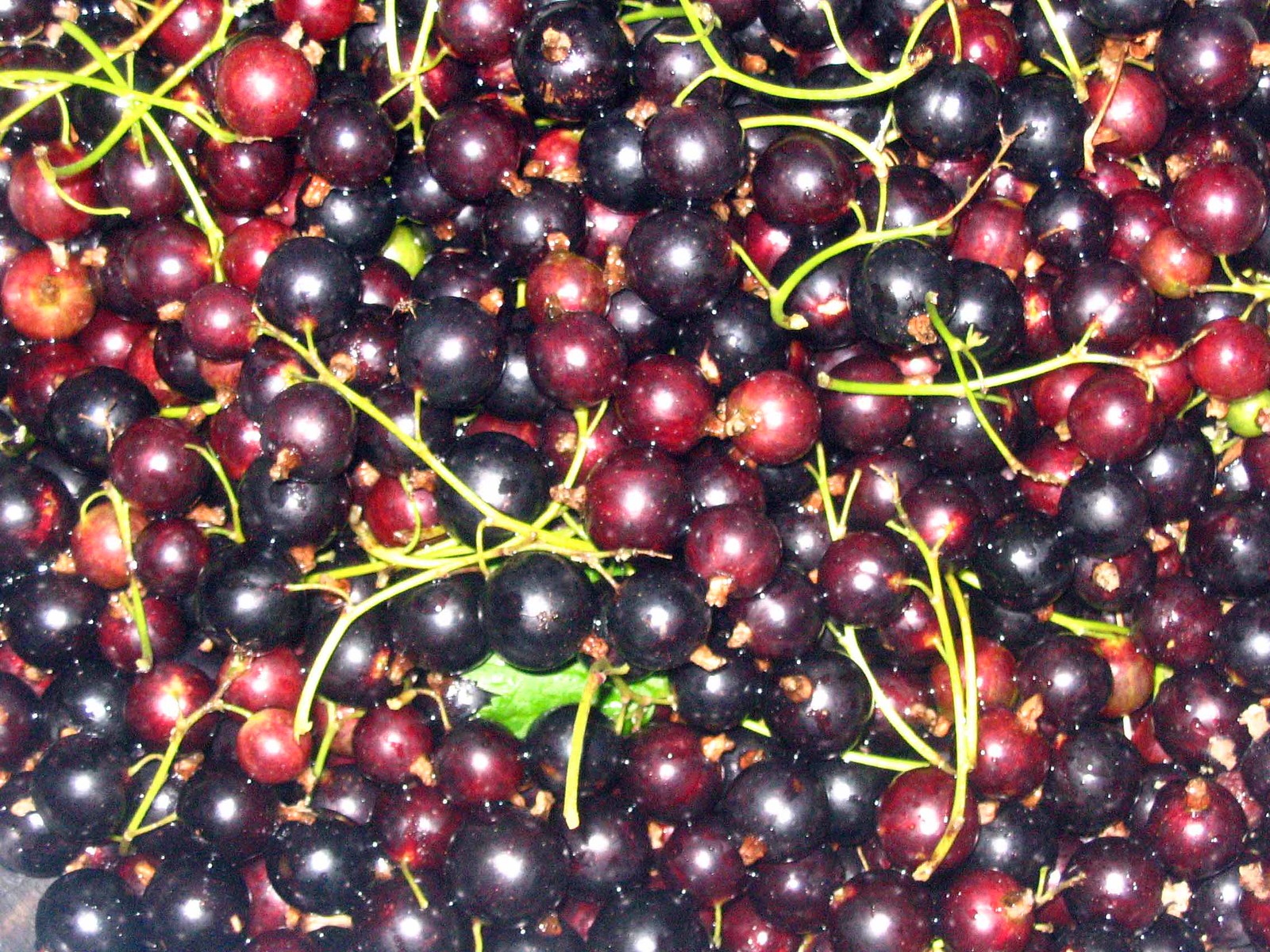This is a detailed photograph of cranberries still growing in a pond. The cranberries, in varying shades of lighter reds, deep reds, to purples, are floating on the water amidst green leaves and stems. The image captures hundreds of these spherical fruits, with some displaying longer stems, particularly the ones in lighter red hues with stems extending about a quarter inch. The stems appear to have been recently picked or stripped, showcasing where the fruits were once attached to the vines. Toward the bottom and middle of the photograph, a green leaf is visible, adding to the natural composition. Overall, the photo presents a vibrant, rich palette of cranberry colors floating together in their natural pond habitat.